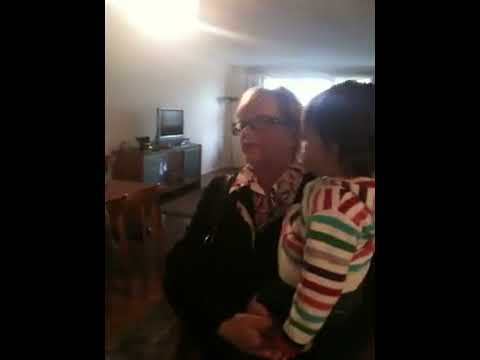In this detailed photograph taken inside a home, a woman with short blonde hair and glasses is seated, cradling a child who appears to be around one and a half to two years old. The woman, who might be a maternal figure, is wearing a dark jacket over a pink and white collared shirt, with a purse draped over her right shoulder. The child she holds has short brown hair and is dressed in a colorful striped sweater featuring shades of green, gold, black, red, and orange over a primarily white shirt. 

The background reveals they are in a room likely serving as a living room, characterized by wooden floors with an area rug and white walls. A dining table with chairs is visible, and a silver TV sits on an entertainment center with cabinets. Additional details include a light source emitting bright white light near the ceiling and vertical black strips flanking the image on both sides. Sunlight streams in through sliding doors, enhancing the cozy and lived-in atmosphere of the space.